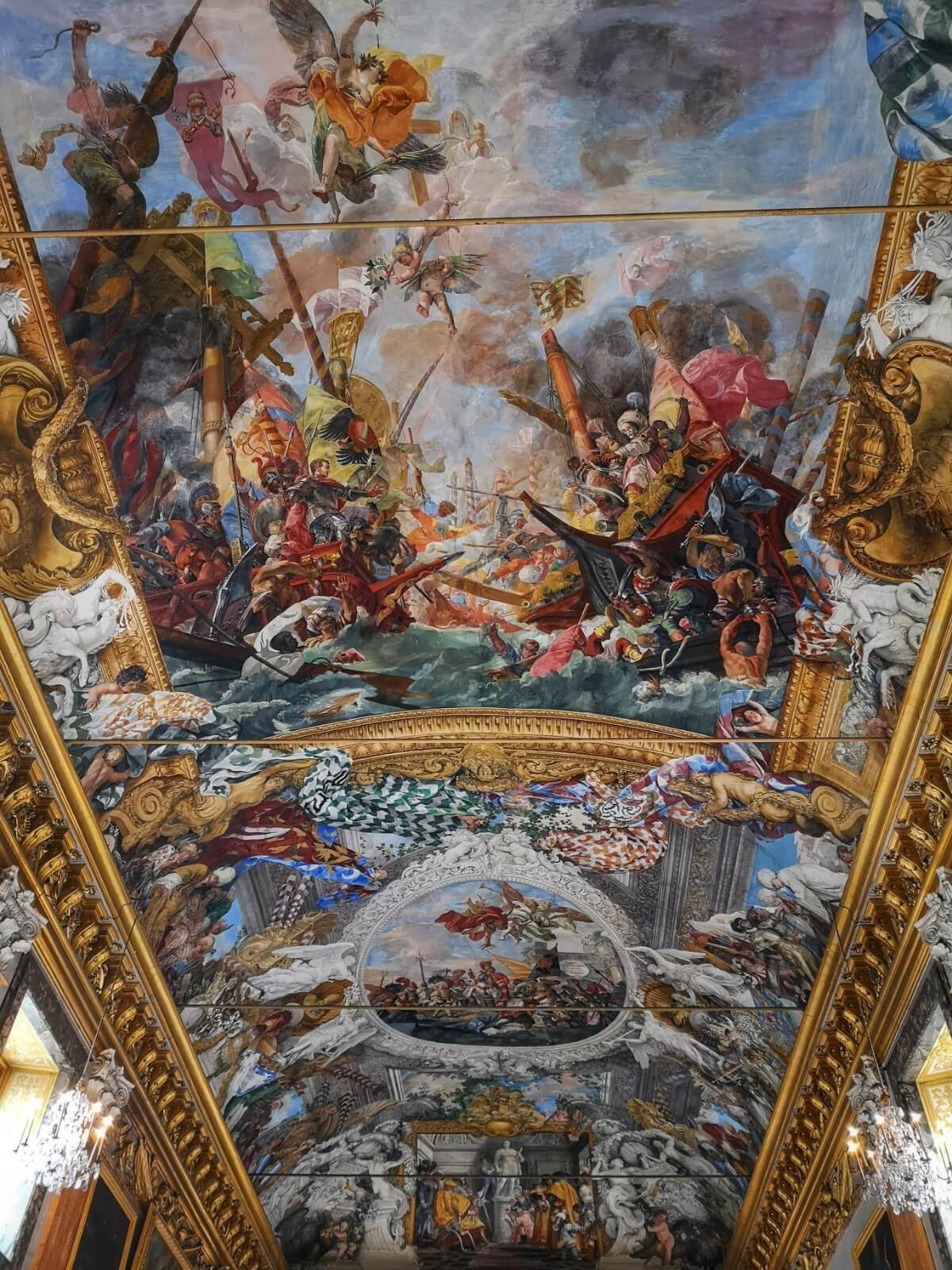This vertical rectangular image captures a detailed segment of a grand mural painted on a curved wall, possibly the ceiling of an old chapel or mansion. The mural, framed by ornate gold borders that extend upwards from the bottom corners, features several continuous sections, each brimming with intricate details. At the topmost portion, flames and wisps of smoke rise into a blue sky, hinting at the chaos of a battle scene below. This battle is set on water, where figures in boats are engaged in combat, surrounded by angelic or divine beings floating above. Descending further, a striking scene unfolds against a vibrant blue background with a prominent white circle at its center, embellished with feathers and surrounded by an array of flying animals. Crystal chandeliers emerge from the bottom corners, adding a touch of elegance to the opulent setting. The mural is a complex tableau of historical and mythical elements, capturing a dramatic narrative in a visually rich, ornate frame.